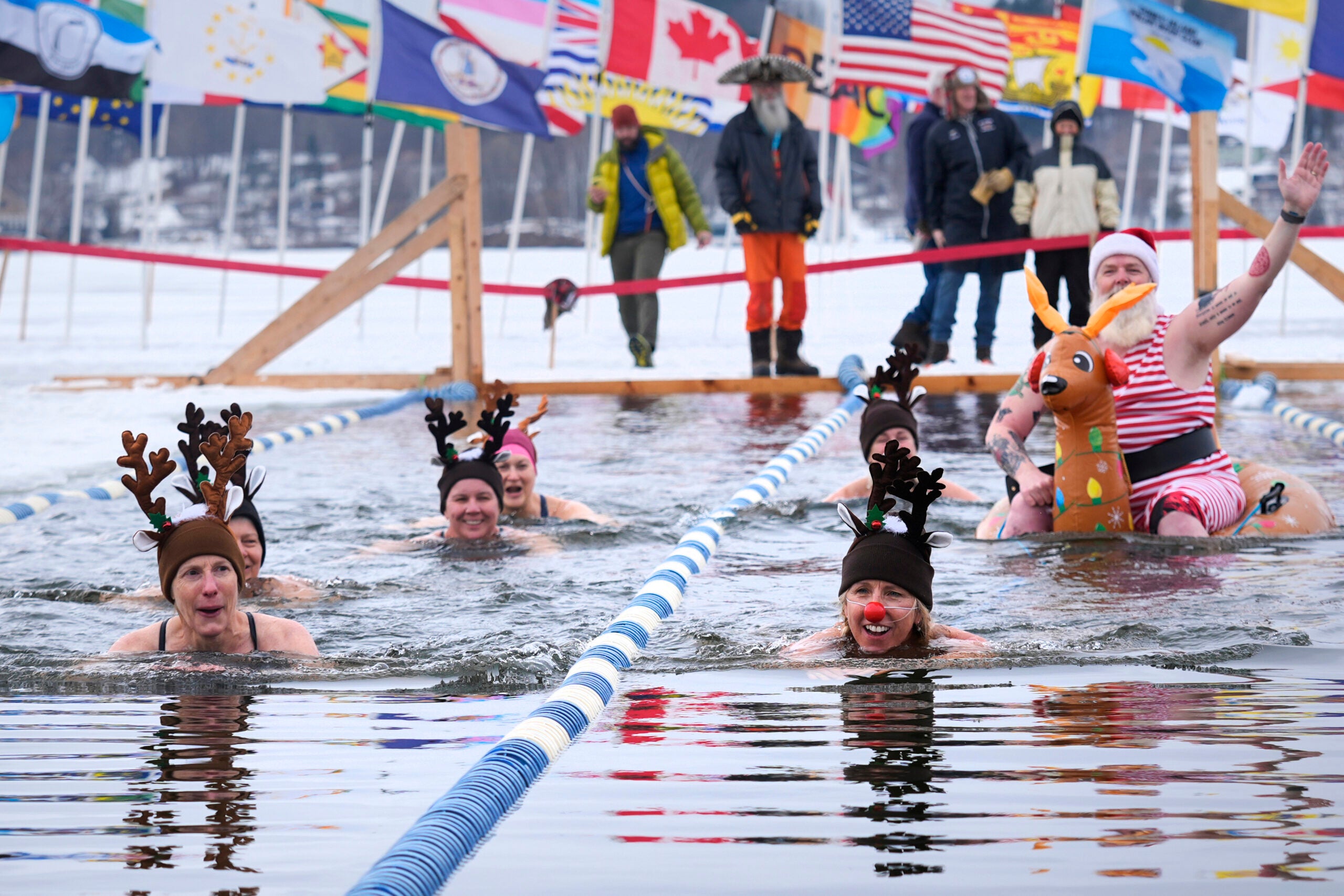This photograph captures the vibrant scene of a whimsical winter swimming event, potentially a race, set in an outdoor pool adorned with blue and white lane markers. The swimmers, predominantly women, are playfully dressed in reindeer hats complete with antlers and red noses, embodying a festive spirit. Adding to the spectacle, a man in a Santa Claus-themed swimsuit—comprising a red and white striped tank top, shorts, a black belt, a Santa hat, and a long white beard—is prominently featured riding an inflatable reindeer with Christmas lights and red earmuffs. He raises his hand, seemingly in joyous acknowledgment. The winter setting is underscored by the blanket of snow surrounding the pool and the spectators clad in heavy winter coats, hats, gloves, and boots. In the backdrop, a diverse array of international flags, including those from Canada and the United States, flutters in the cold air, hinting at an international competition or festival. The overall mood is cheerful, with the participants’ smiles and the onlookers’ attentive presence painting a picture of communal celebration amidst the chill of winter.